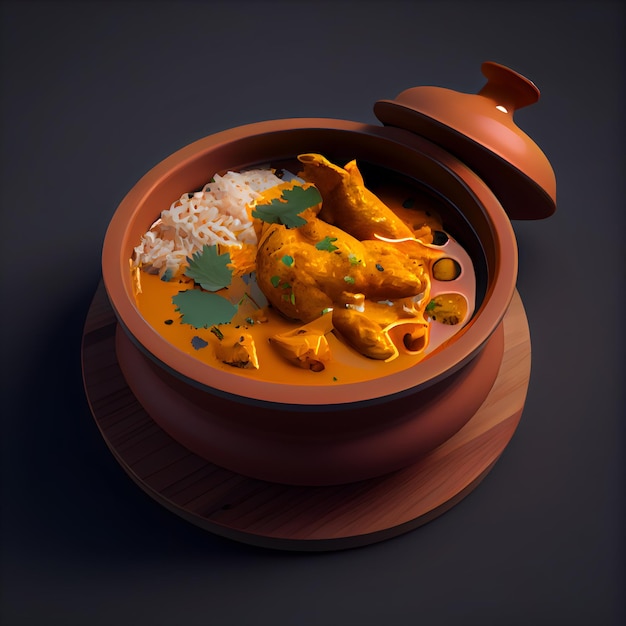The image presents a tantalizing culinary scene, showcasing a square composition dominated by a dark charcoal background. At the heart of the image, a wooden plate cradles a rustic terracotta casserole dish, adding a touch of warmth and homeliness. The casserole’s lid is artfully positioned, leaning against the dish's upper right corner, inviting curiosity about the delightful contents within.

Inside the dish, a vibrant curry and rice medley beckons the viewer. Succulent chicken pieces are nestled amidst the robust curry, their golden brown hues contrasting beautifully with the rich sauce. A portion of fluffy white rice resides in the top left corner of the casserole, punctuating the dish with its simplicity. Garnishing the ensemble, a few delicate flakes of parsley are scattered, adding a fresh, green flourish.

Upon closer inspection, however, the image exudes an uncanny quality; the elements appear almost too perfect, suggesting it may have been generated by AI, lending an intriguing, surreal touch to this otherwise mouthwatering portrayal.